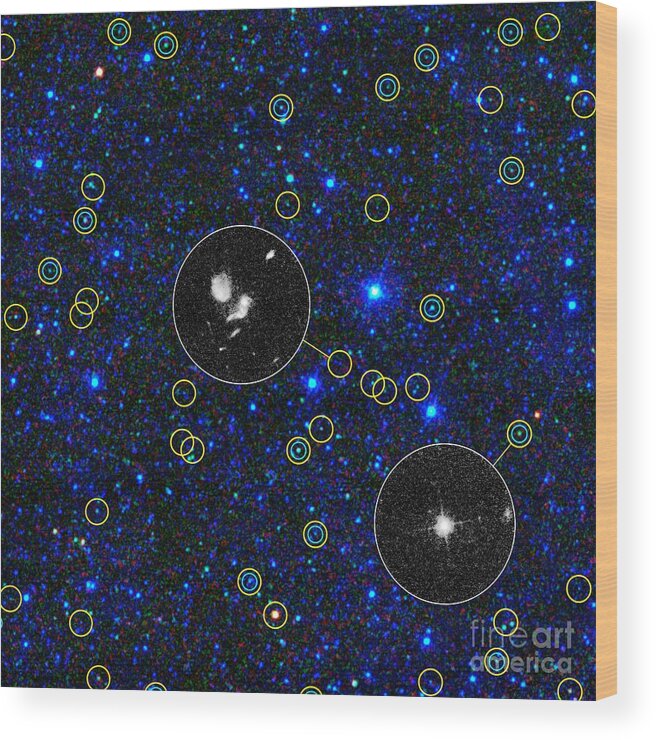This detailed artwork appears to be a digitally generated image printed on a wooden plaque, showcasing a night sky teeming with celestial bodies. The predominantly black sky is interspersed with numerous blue dots and bright yellow circles, some of which are a combination of yellow and blue. On the right edge, you can glimpse the side of the wood, emphasizing its three-dimensional nature. Two significant yellow circles are highlighted with insets that are magnified to display what seems to be photographs of stars or star systems, suggesting a guided diagram or a telescopic map of the night sky. The piece includes a watermark in the bottom right corner that says "Fine Art America," marking it as a fine art print. The blue, black, and yellow color scheme, along with meticulously marked celestial points, indicates the artist's keen interest in astronomy and space, creating a visually compelling piece for star enthusiasts.